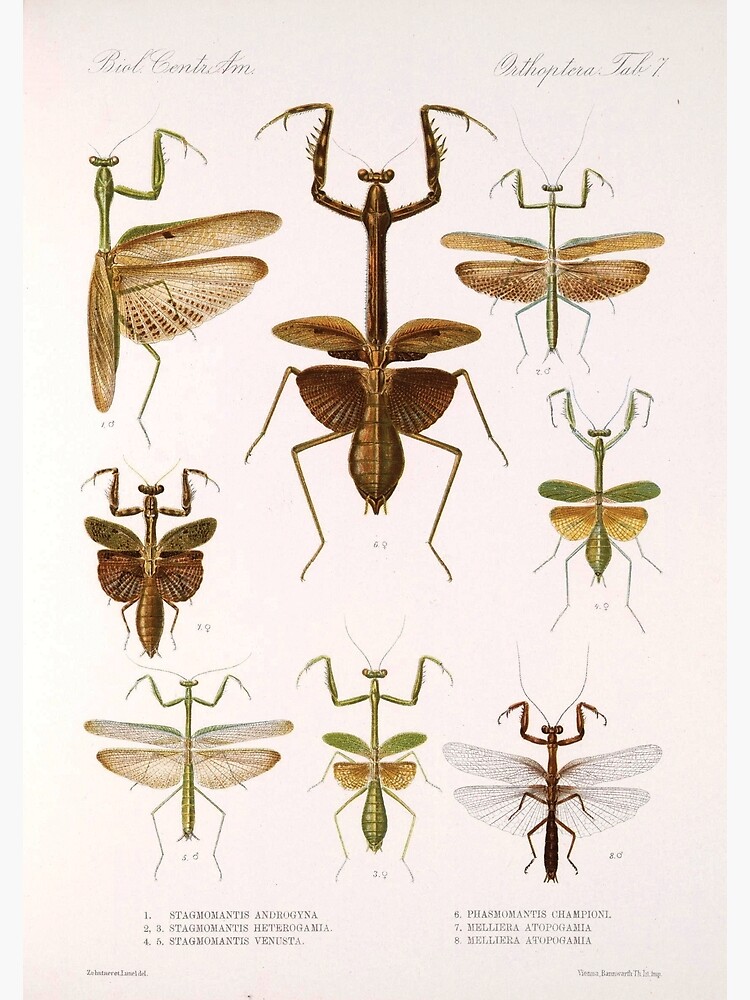This vertical portrait layout illustration features a cream-colored or off-white background, resembling an old educational plate. It showcases eight different variations of praying mantises. Across the top in faint, cursive italic font, likely their scientific names, are inscribed in hard-to-read black text. The mantises are arranged in three rows, with sizes varying such that the largest is centrally placed in the top row, flanked by smaller ones. The following rows continue with similar placements, leading to a uniform size in the bottom row. The insects are predominantly in shades of brown, yellow, and green. At the bottom, the page includes two numbered columns of text, one to eight, providing names and descriptions of each mantis type in similarly difficult-to-decipher black font. The detailed and antique style underscores the diagrammatic, descriptive nature of this entomological artwork.